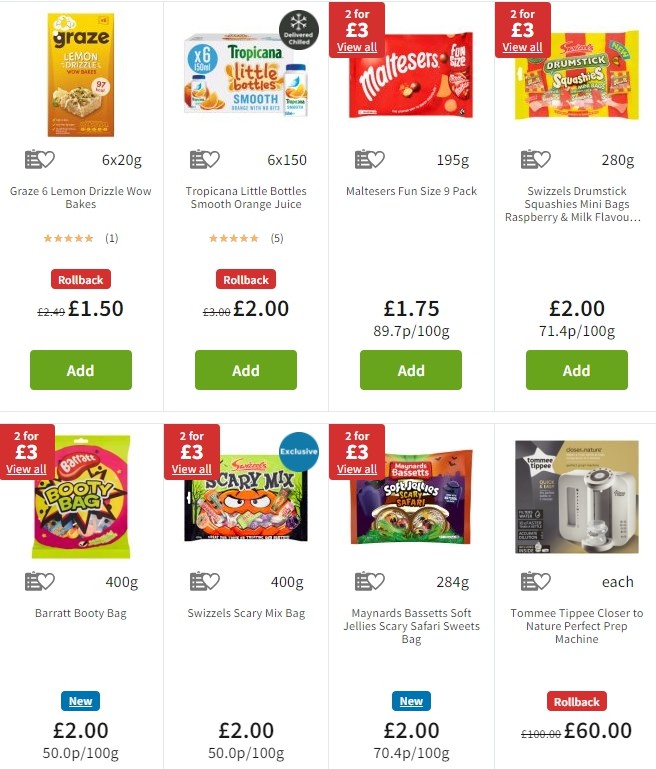The image showcases a detailed webpage from a retail site predominantly offering food items. At the top of the page, a package of baked goods labeled "Graze 6 Lemon Drizzle Wild Bakes" is prominently featured. Accompanying this are several other food products, each represented with their own picture. 

Beside the baked goods, an item named "Tropicana Little Bottles Smooth Orange Juice" is displayed, featuring a clear image of the juice bottles. Adjacent to this is a red package labeled "Maltesers Fun Size 9 Pack", which appears to be a pack of fun-sized chocolate candies. 

Continuing along the row is the "Wizzles Drumsticks Squashies Mini Bags, Raspberry and Milk Flavored", presented in a bright yellow and red package, suggesting a fruity candy variety. 

In the bottom row, there is a "Barrett Booty Bag", likely another candy product, followed by "Skix Wizzles Scary Mix", which appears to be a mixed candy assortment. Further down the line, the "Maynards Bassets Soft Jellies Scary Safari Sweets Bag" is displayed, another candy item designed with a playful theme.

On the far right of the selection, diverging from the food items, is a kitchen appliance named "Tommy Tippy Closer to Nature Perfect Prep Machine", hinting at its function as a food preparation device designed for convenience in the kitchen.